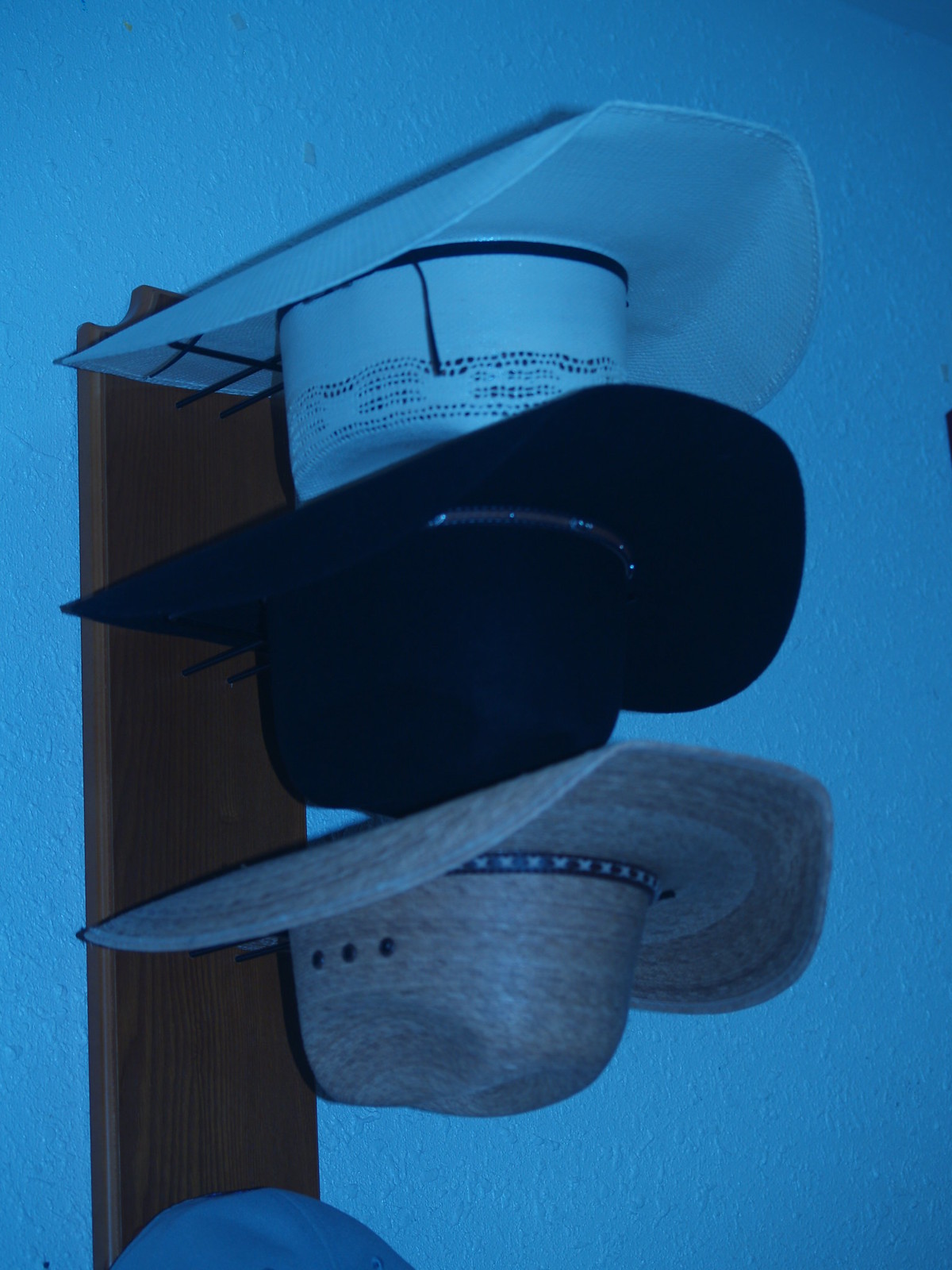The image depicts three distinct cowboy hats hanging upside down on a brown wooden hanger attached to a wall that appears blue, either due to paint or lighting. The hanger supports these hats using black metal rods. The upper hat is white, accented with a black band and an open circular pattern around the top. The middle hat is black, adorned with a light brown band, with its brim slightly folded. The bottom hat is gray-brown, resembling a straw texture, featuring a black band with a white repetitive dot pattern and three circular beads on its side. A portion of a possible fourth hat or an item, made of gray cloth-like material, peeks out at the very bottom of the image.